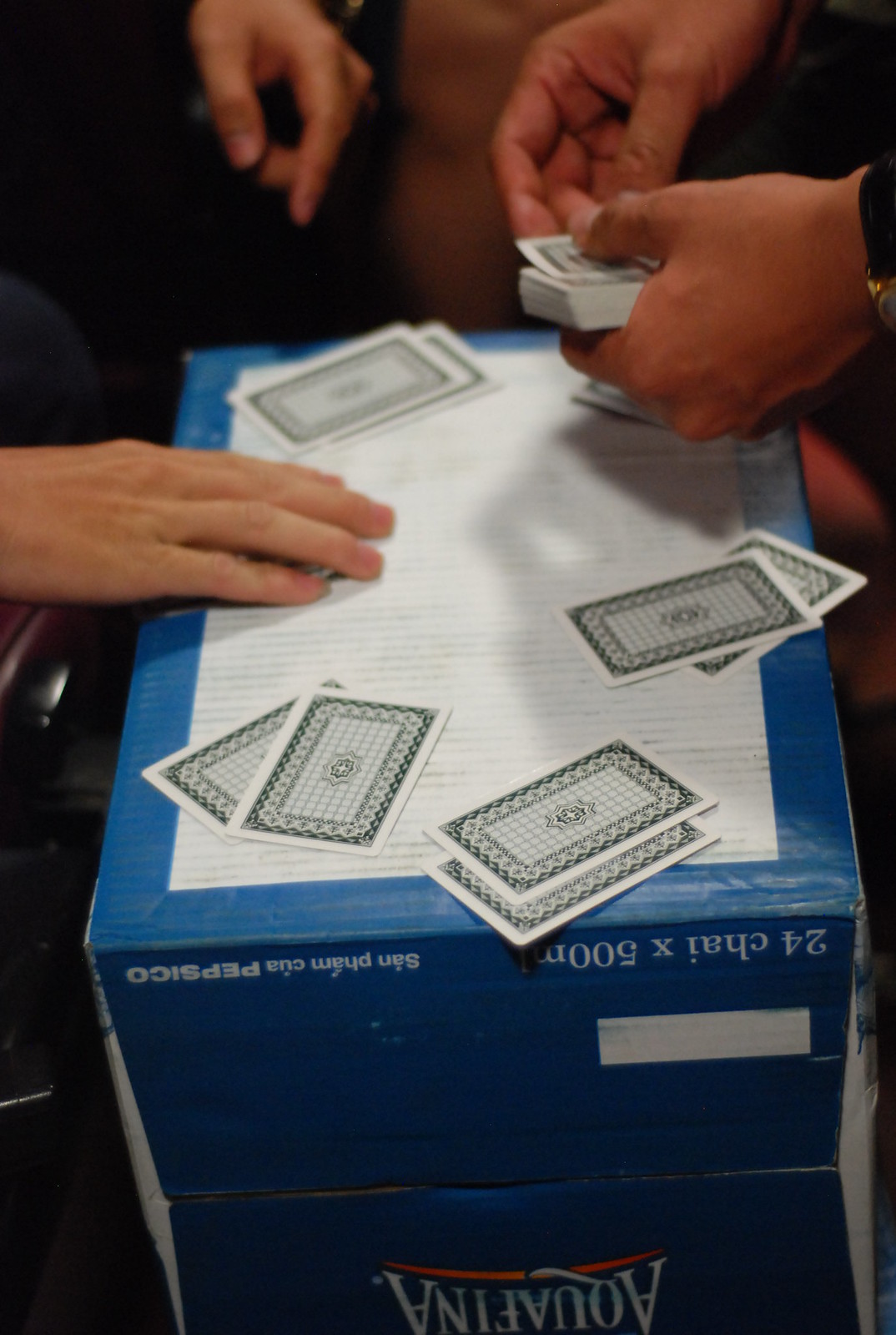In this photograph, we see an intimate scene of a card game in progress, captured with a focus on the action at hand. The playing surface is an inverted cardboard box, initially used for Aquafina bottled water, as indicated by the recognizable upside-down logo near the bottom of the image. The makeshift table's resourcefulness adds a casual, improvisational charm to the scene.

Two pairs of hands dominate the frame, with the players' identities remaining anonymous. The hands on the right, belonging to a person who appears to be either dealing or preparing to draw a card, grasp a deck firmly, with the right hand poised to lift the top card. Conversely, the hands on the left, also engaged in the game, mirror their opponent's focus and intensity. The image's tight crop emphasizes the interaction between the cards and the players, omitting any facial features or gender identifiers, thereby universalizing the depicted moment.

Four distinct piles of two cards each are strategically placed on the cardboard box: one at the top, another towards the bottom left, a third positioned at the bottom right, and the last one lying centrally on the right side. The arrangement of these piles suggests an ongoing game strategy, inviting viewers to ponder the potential moves and winner in this engaging snapshot of leisure and competition.